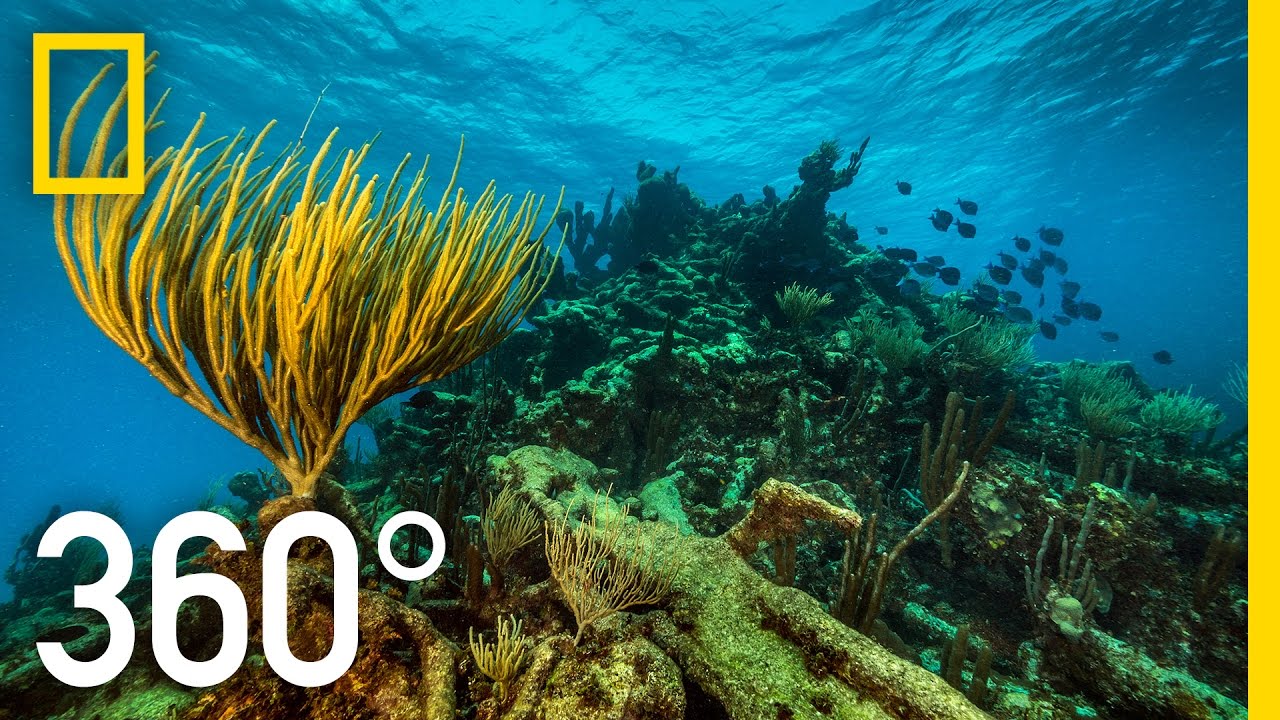The image is a professional underwater shot likely taken by National Geographic, as indicated by the signature yellow rectangular outline in the upper left corner and a yellow bar down the right side. Prominently displayed in large white text in the lower left corner is "360 degrees," hinting at the immersive nature of this visual experience. The scene unveils a vibrant underwater world where the clear blue water allows light to illuminate a striking composition of underwater vegetation. Centered in the image is a large golden-brown plant, resembling a sea tree or bush, accompanied by smaller baby plants at its base. This lush plant life is situated on a mound that gently inclines upwards, showcasing various green and dark green plants interspersed possibly with coral. At the top right of this mound, a school of small fish swims gracefully, adding a dynamic element to the serene underwater landscape. The surface of the water is visible above, where light filters through, enhancing the clarity and depth of this captivating underwater scene.